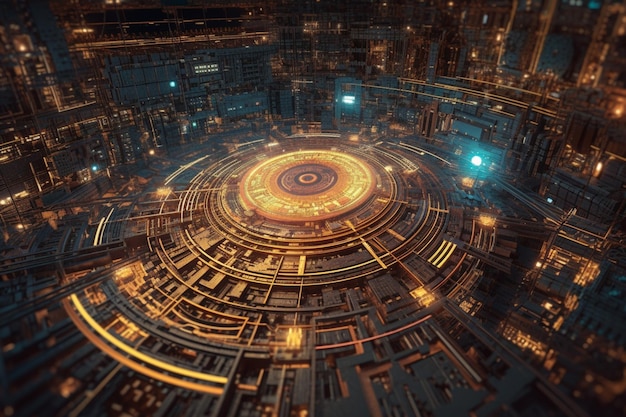The image appears to depict the intricate interior of an advanced piece of technology, potentially an AI-generated visualization or a sci-fi spacecraft interior. Dominated by dark, predominantly black backgrounds, the composition features a multitude of finely detailed components rendered in a navy blue hue, likely a result of the image’s lighting rather than their actual color. Central to the image is a prominent circular object emitting a radiant, warm yellow light. This central hub is surrounded by concentric rings, which contain various technological elements resembling lines, wires, sections, and compartments. The yellow center is further accentuated by additional rings of varying sizes and colors, including bluish-orange and smaller orange bands. Bright blue lights sporadically illuminate the scene, with a noticeable light on the right side and another in the background. The overall structure, extending upwards in repetitive patterns akin to stacked stories, evokes the complex, futuristic aesthetic of a spacecraft or a mesmerizing element from a sci-fi universe, complete with an enveloping back wall that ties together the technology-laden environment.